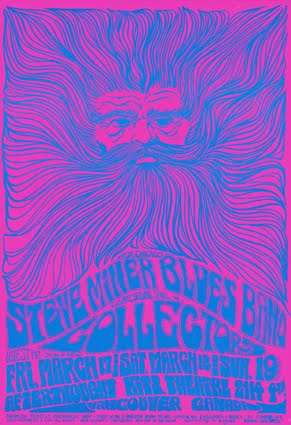The image is a visually striking poster featuring a central figure, appearing to be a king-like man with a mustache and beard that fan out in a large square pattern around his face. His face, colored in bright pink, stands out prominently against the vibrant background. The poster predominantly showcases neon blue and pink hues, adding to its eye-catching appeal. The top of the poster displays the man's face, with detailed features including his forehead, eyebrows, eyes, and nose, but his chin remains obscured within the pattern of the mustache and beard.

Additionally, the poster includes significant signage with an array of text that reads: "Steve Minor Blues Band Collectors" followed by event dates "Friday March 17th, Saturday March 18th, Sunday the 19th". There are also more words in blue bubble text, indicating further details. The vibrant neon colors, including light blue streaks and bright pink elements, enhance the overall artful and electric design of this poster.